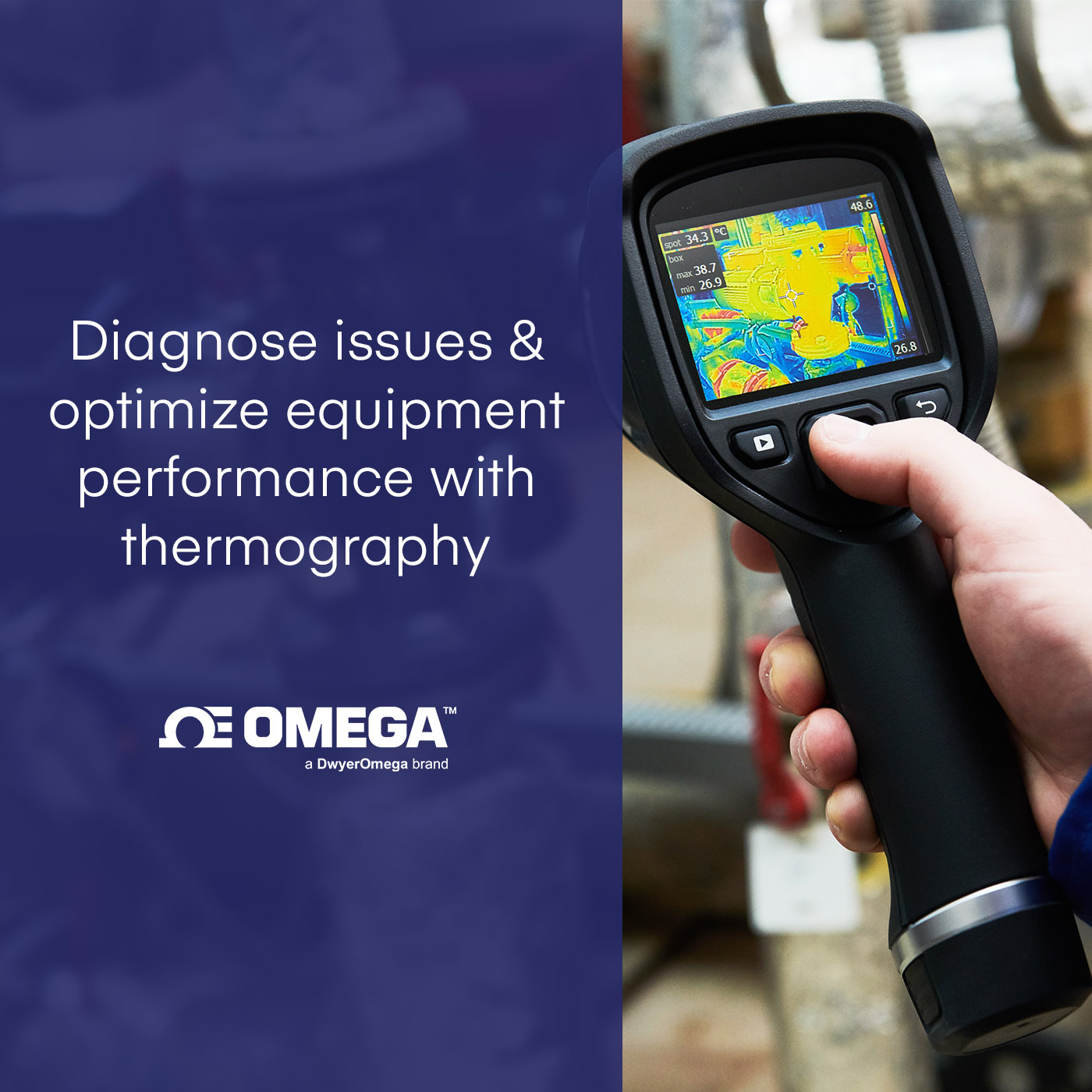This image serves as an advertisement and instructional guide for using a thermography device, branded under Omega, a Dwyer Omega Brand. The image is divided into two primary sections. On the left, a blue overlay features the Omega logo—composed of the Omega symbol integrated with an 'E'—and the tagline "Diagnose issues and optimize equipment performance with thermography" in white font. The background has some indistinct images, adding a technical ambiance.

On the right side, a person is holding the thermography device, which is black with a handle resembling a small flashlight or a pole. The device has an LCD screen displaying thermographic readings in neon colors—primarily blue and gold. The screen interface includes numerical readouts and other indicators for thermographic data. The user’s thumb is centered on the device, likely interacting with a central control button. Additional buttons are visible: one to the left, marked by an arrow, and another to the right. A silver band encircles the handle, adding a design detail to the predominantly black device. The background is blurred, with unidentifiable shapes, focusing the viewer’s attention on the device and its usage.